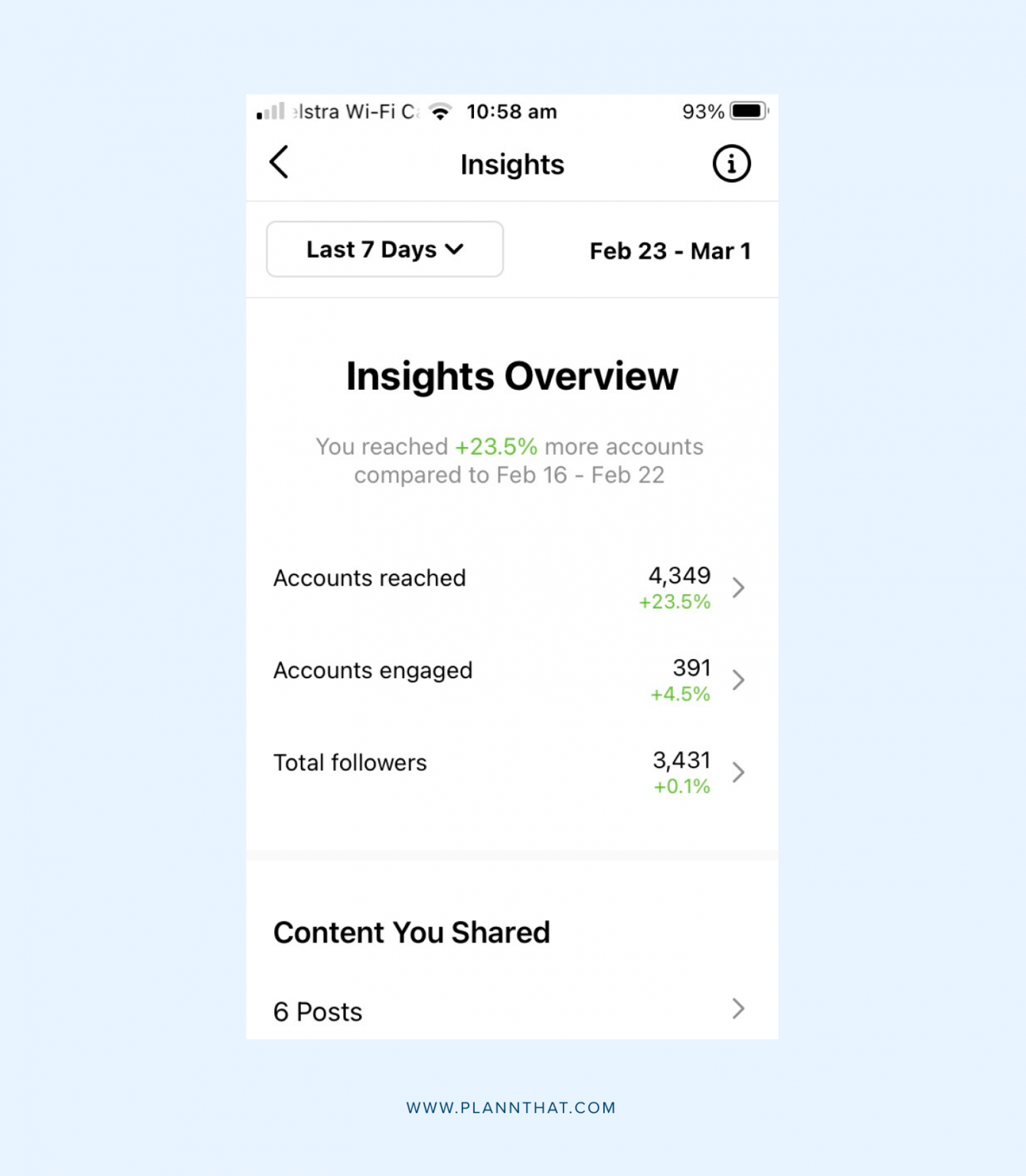This is an image of an iPhone displaying a website, with the device's status details clearly visible. The battery life is at 93% and the time is 10:58 AM. The Wi-Fi icon indicates a semi-strong connection, though part of the Wi-Fi status text, displayed in light grey on the left side, is partially obscured. At the top of the webpage, the title "Insights" is displayed in black, accompanied by a left-pointing arrow on the far left and an information icon (a circle with an "i" in the middle) on the far right. 

Below this header is a section where "Last 7 days" is selectable via a drop-down arrow, located inside a box, next to the date range "February 23rd to March 1st" on the right. In the main body of the page, a prominent heading reads "Insights Overview" in black text, followed by a smaller subheading stating "You reached 23.5% more accounts compared to February 16th to February 22nd." 

The page proceeds with detailed metrics:
- "Accounts Reached" shows 4,349, which is an increase of 23.5%, illustrated with a right-pointing arrow.
- "Accounts Engaged" lists 391, up 4.5%, highlighted in green along with a right-pointing arrow.
- "Total Followers" notes 34,031, reflecting a 0.1% increase, again marked with a right-pointing arrow.
- "Content You Shared" reports six posts, with an associated right-pointing arrow.

The bottom of the webpage features a light blue border, within which the URL "www.planthat.com" is displayed.